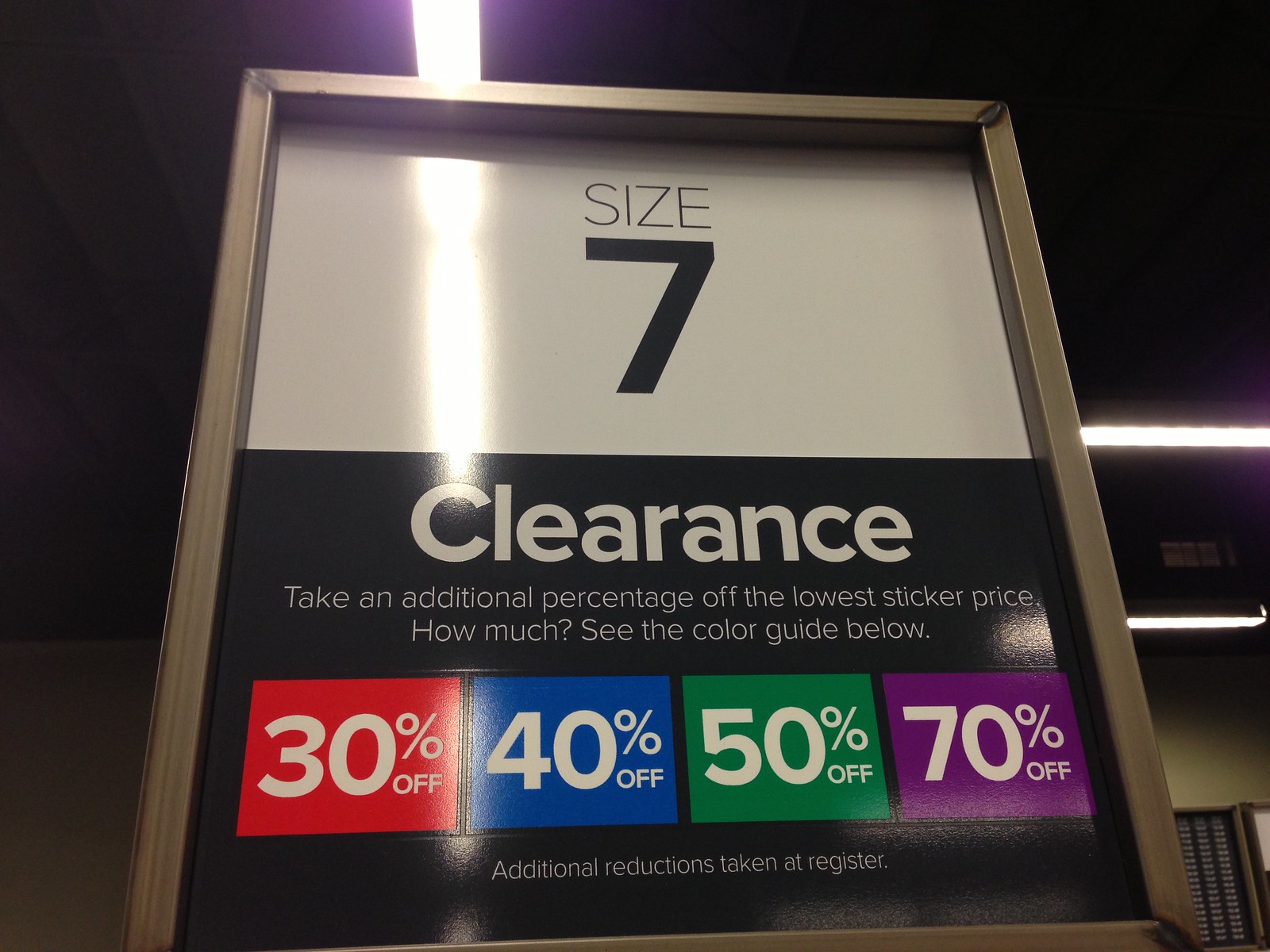This image captures a clearance sign prominently displayed in a retail store. The sign is framed with a dark gray or bronze metal border, and its design is split into two sections. The top half features a white background with the text "Size 7" in bold black letters. Below this, the black background showcases the word "Clearance" in large white letters, followed by the phrase "Take an additional percentage off the lowest sticker price. How much? See the color guide below." The color guide is listed in four colored boxes: red (30% off), blue (40% off), green (50% off), and purple (70% off), each indicating the discounts available. The phrase "Additional reductions taken at the register" is also included in white text. The store environment hints at a shoe store, with storage and a door in the background. Overhead, white fluorescent lights reflect off the sign, contributing to the illuminated setting. The grayish wall and a blue-shuttered window to the right add subtle details to the overall scene.